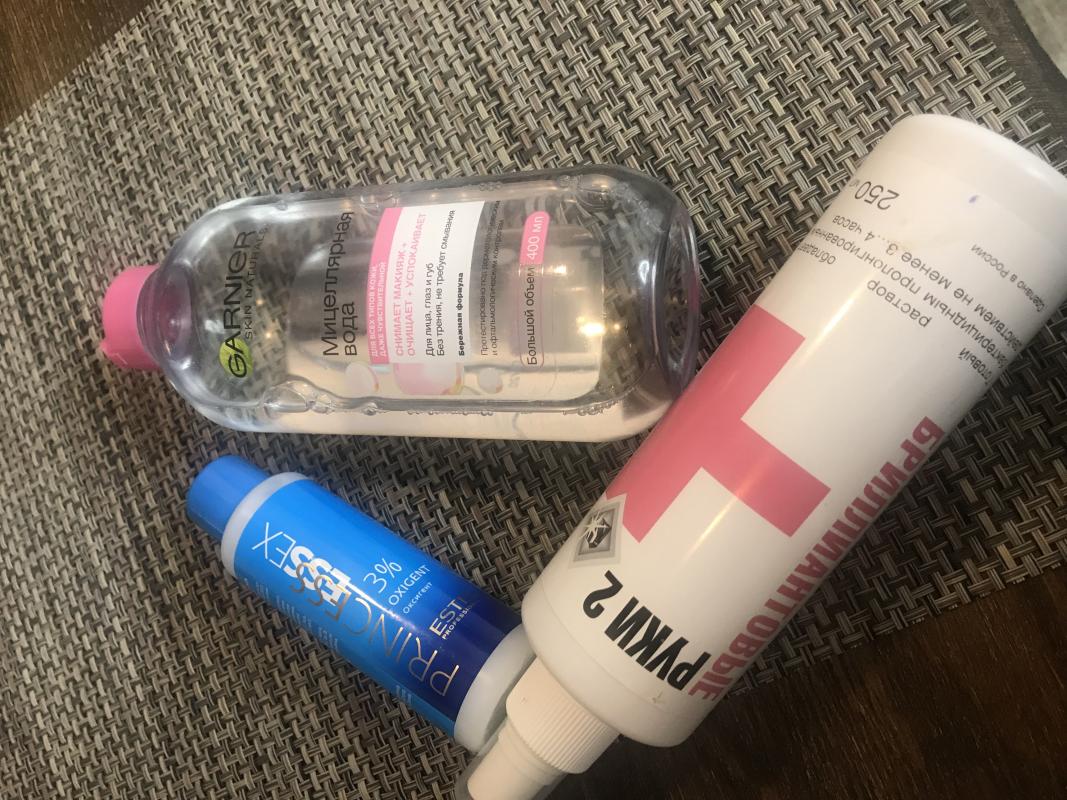The image showcases three distinct bottles, each appearing to serve different purposes. The first bottle is blue, prominently featuring the text "3% Oxygen" and "Princess OxyCream," suggesting it may be a product related to skincare or haircare, possibly a facial cream or hair treatment. The next bottle is a clear plastic container with the label "Garnier," followed by non-English writing. The liquid inside seems thick, resembling either castor oil or baby oil. The third bottle is a spray bottle with what seems to be non-English characters resembling "P-Y-K-N-2." Adorned with a red cross, this bottle could be associated with first aid. All these items rest on a professionally woven mat, providing a rustic background that enhances the aesthetic appeal of the scene.